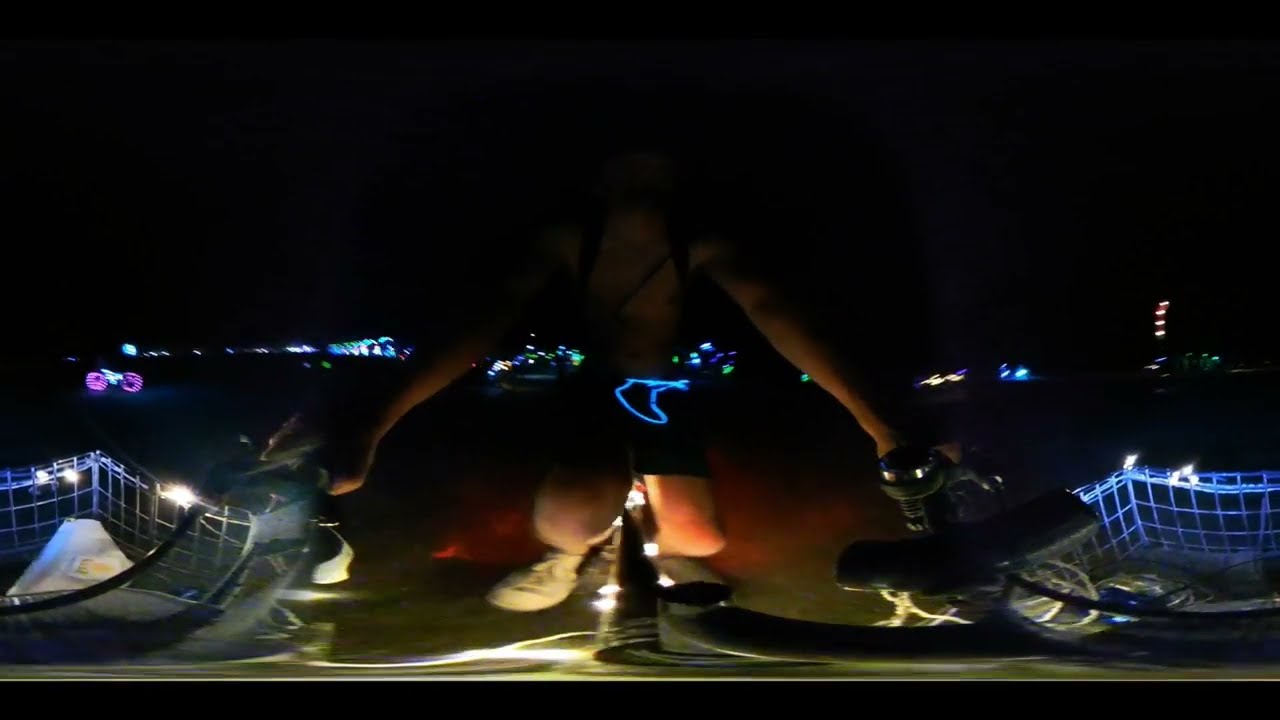The rectangular illustration features a man, who appears to be white, riding a bicycle in an indoor cave-like setting with a large rock wall and a dark opening in the background. The scene is distorted in a way that the handlebars and the baskets of the bike appear duplicated on both sides, despite the single man centered in the image. He is shirtless, wearing only black shorts with a blue waistband, and a backpack with visible black straps. The man is gazing upward and to the side. The ground beneath him resembles yellowish-gold sand, adding to the cave-dune atmosphere. Surrounding him are some stand lights, with additional scattered people, some on bicycles, illuminated by these lights. The image has a dark ambiance, with central and right-hand light sources contributing to the scene’s dramatic lighting.